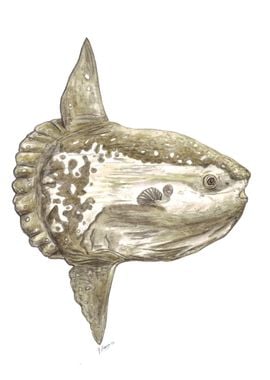This image features an abstract, antique-style painting of a fish fossil, centrally positioned against a white background. The fish appears to be made of a brownish, stone-like material, with two distinct fins—one dorsal and one ventral—painted in a gray hue. The fish head, which resembles something that might be mounted on a wall, shows an open mouth and a visible right eye with a horizontal white stripe extending from its neck to its eye. The body of the fish is lighter in the middle, adorned with white patches and brown spots. Uneven, scalloped protrusions at the back suggest a shell or vertebrae-like structure. The artwork is marked with an unreadable signature at the bottom, enhancing its abstract quality.